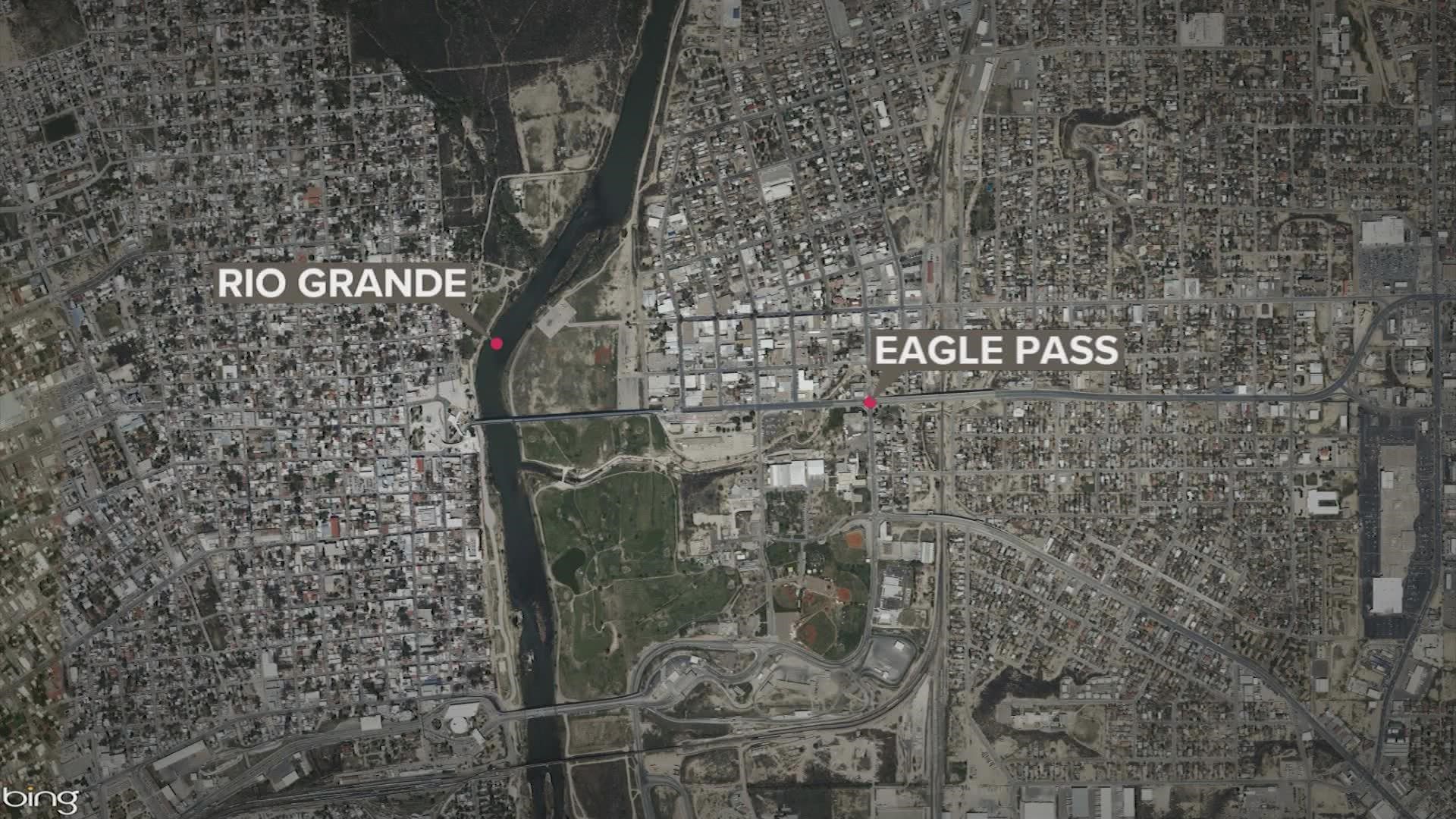In this bird's-eye view map, a satellite image showcases a city bisected by the Rio Grande river, flowing vertically down the center. On the left side of the river, near the bottom left corner, is a watermark with the text "Bing" in white. The river itself is labeled "Rio Grande" with an arrow pointing to a circular dot in the water. East of the river, a dot marks an intersection labeled "Eagle Pass." The landscape on both sides of the river is densely populated with residential buildings and housing districts, appearing as clusters of squares typical of an aerial city view. Additionally, there are three bridges visible near the southern part of the river, connecting the two sides of the city.